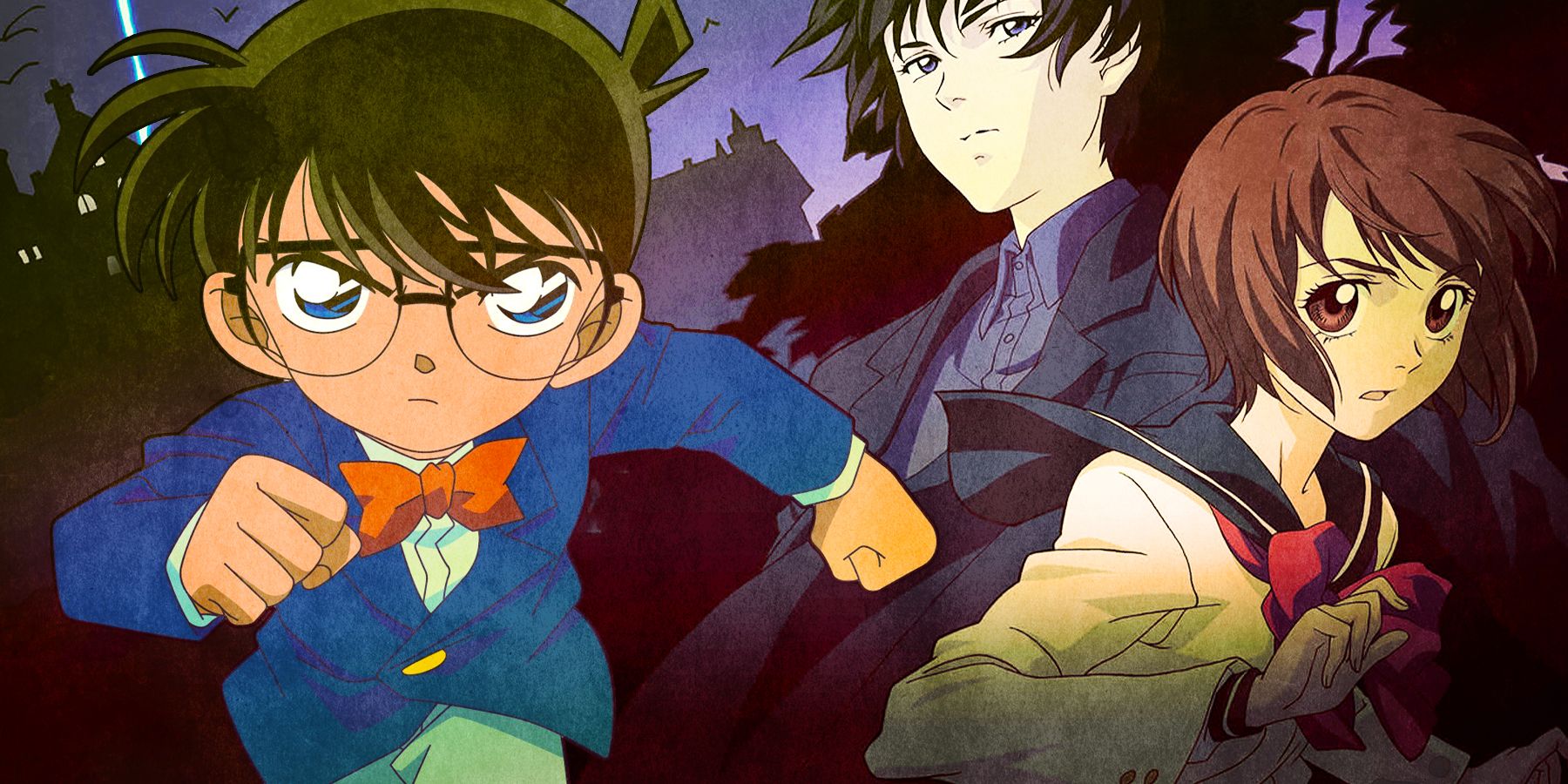This anime-style illustration vividly depicts a trio of characters, each showcasing a resolute or contemplative expression, set against a dark, eerie backdrop that includes a purple-tinted building resembling a church or haunted house. Dominating the left side, a young boy or man with brown hair and large eyes charges towards the viewer, wearing a blue blazer, brown bow tie, and 80s-style glasses, exuding determination. On the right, two characters are positioned back-to-back: a young woman with short brown hair is adorned in a white school uniform with red and navy accents, including a red scarf and black cape, her face etched with fear. Behind her stands a young, pale man with black hair, dressed in a dark jacket and blue shirt, radiating a mysterious aura. The intricate details and contrasting emotions of the characters heighten the intensity and depth of the scene.